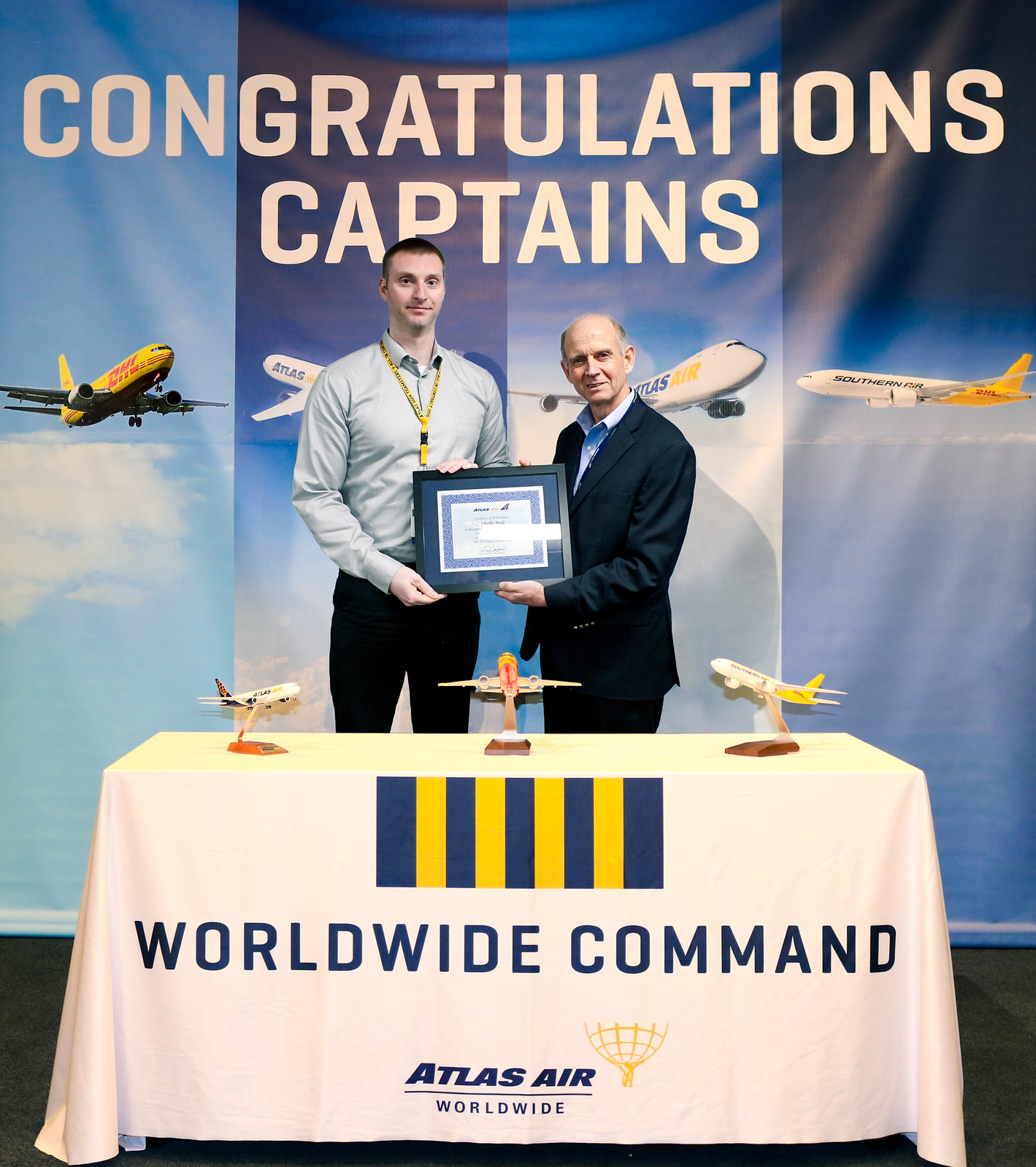In this detailed image, a person is receiving an award certificate from another individual, set against the backdrop of a large banner featuring four panels each depicting a plane flying in the sky. Prominently displayed on the banner in large white letters are the words "Congratulations Captains." One of the planes has "Atlas Air" on its side and another is labeled "DHL." In front of this banner stand two men, both holding up a framed certificate with a blue matting. The person on the left is tall and young, with short brown hair, wearing a gray button-up shirt and black pants. The person on the right is older and mainly bald, donning a blue suit jacket with a lighter blue shirt. In front of them is a table covered with a white tablecloth, adorned with three model airplanes. Below the table, large blue letters spell out "Worldwide Command," accompanied by the Atlas Air Worldwide logo, featuring a figure shouldering a globe.